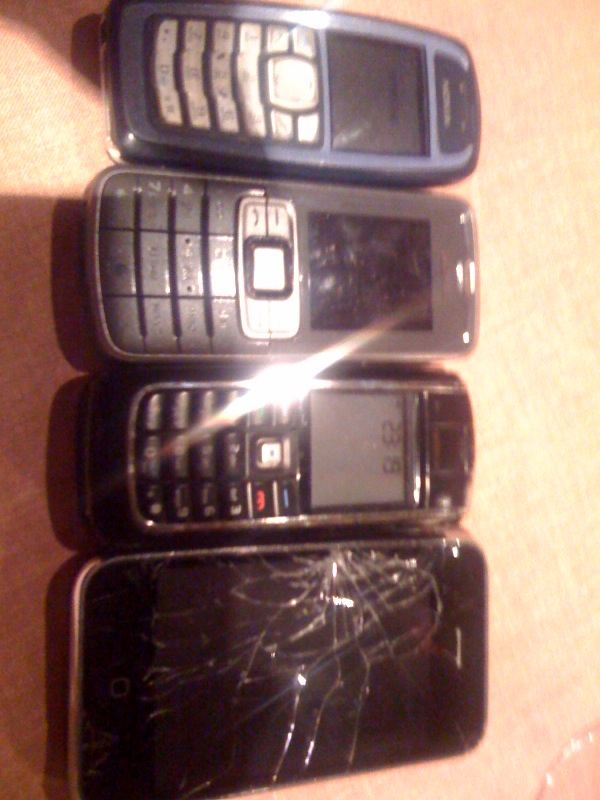This image presents four cell phones arranged vertically on a tan table. The first three phones are older models possibly dating from the 90s or 2000s, while the fourth phone is a modern smartphone with a shattered screen. 

The first phone features a blue casing with silver buttons and appears operational, as the screen shows some text. The second phone is dark gray with silvery buttons, though the screen is obscured by reflected light. The third phone is black with a silver button layout and a screen displaying the number "2319." Reflective light also creates a shine on this phone, particularly on its right side.

The fourth and newest phone is entirely black and touchscreen, but its screen is severely cracked, contrasting with the intact condition of the older phones.